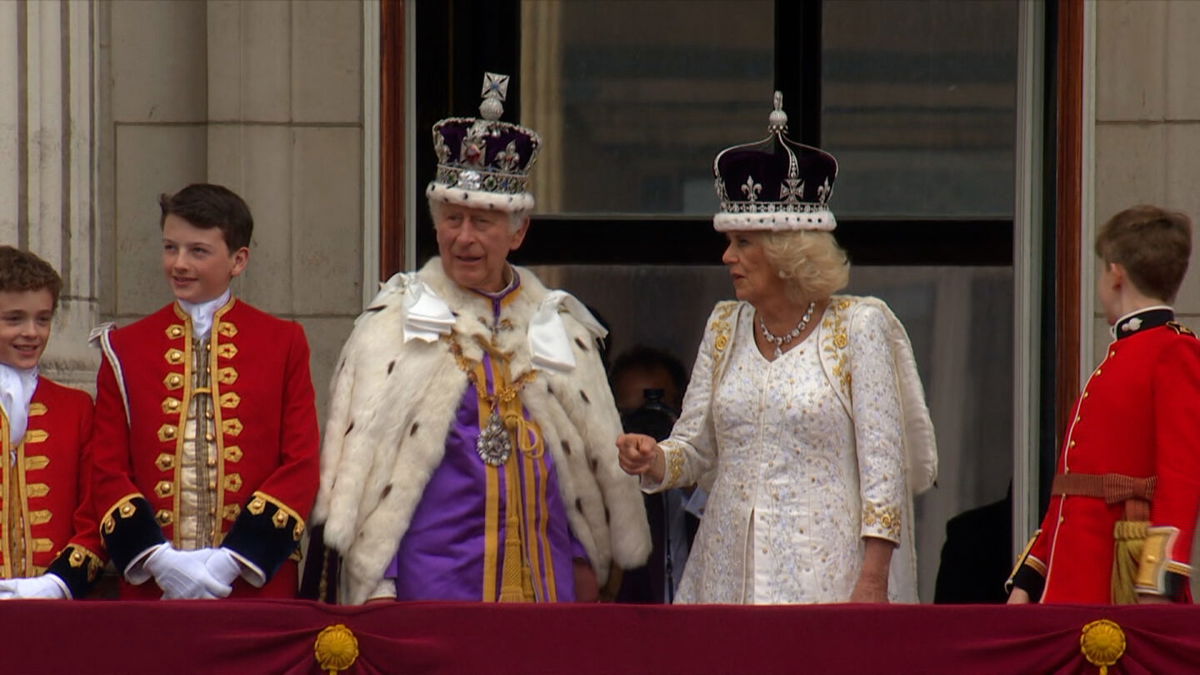The image depicts a royal scene featuring Prince Charles and Camilla, both adorned in regal attire and elaborate crowns. Prince Charles, positioned on the left, dons a plush, fur-trimmed royal jacket with purple hues accented by stripes of orange. Complementing his opulent ensemble is a large, heavily decorated crown with a fluffy base, emphasizing his majestic presence. Standing beside him, Camilla is elegantly dressed in a flowing white gown embellished with golden embroidery. Her crown, similarly ornate with a white base, rests atop her blonde hair. Together, they are the focal point amid a backdrop of young boys, likely aged 10 to 15, dressed in red royal suits with golden buttons and white gloves. The scene is set on a balcony, adding to the grandeur, with photographers and various onlookers capturing the moment. Additionally, a maroon tapestry drapes at the bottom of the scene, further enhancing the rich and regal atmosphere.